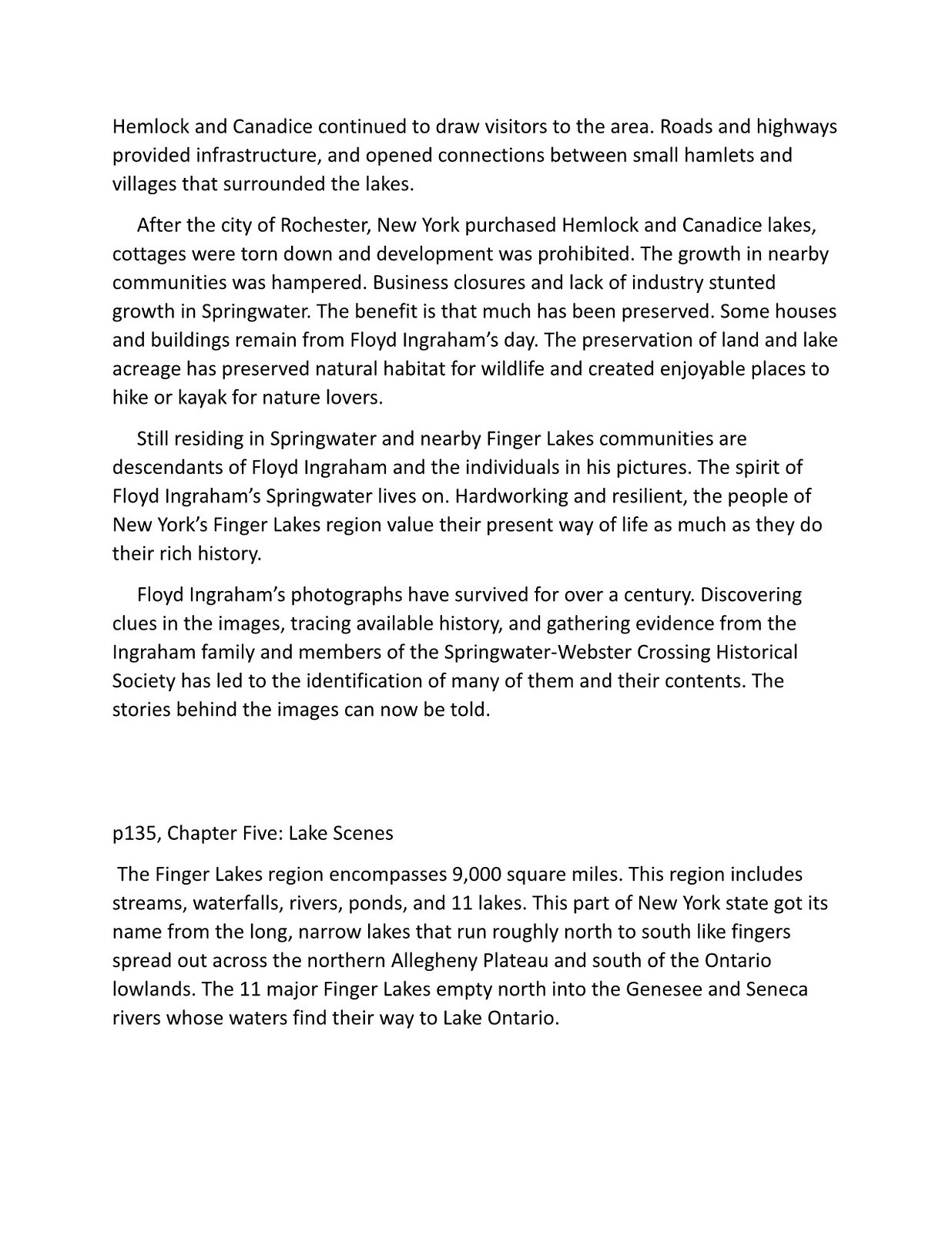The image depicts a white page filled with 8-point font text, apparently from a book, specifically from page 135 in chapter 5, titled "Lake Scenes." The content focuses on the Finger Lakes region of Upstate New York, encompassing 11 long, narrow lakes that collectively cover 9,000 square feet and are renowned for their scenic beauty and historical significance.

The text describes how Hemlock and Candace lakes (sometimes referred to as Canada's) continue to attract visitors, benefiting from modern infrastructure that connects small hamlets and villages around the lakes. However, development around these lakes was restricted after the city of Rochester, New York, purchased them, leading to the demolition of numerous cottages and a halt in further development. This had the effect of slowing growth in nearby communities such as Springwater, resulting in business closures and a lack of industry. On the positive side, this preservation effort has maintained much of the natural habitat, making the area a haven for wildlife and a popular spot for hiking and kayaking.

The narrative also touches on the historical and cultural legacy of Floyd Ingram, whose photographs from over a century ago have been crucial in tracing the region's history. Many of these images have been identified and cataloged through the efforts of the Ingram family and the Springwater-Webster Crossing Historical Society. Floyd Ingram's work is celebrated for capturing the spirit of the area's resilient and hardworking residents, many of whom still live in Springwater and other nearby Finger Lakes communities. The preserved landscapes and historical structures tell the story of a region that values its rich past while embracing its present way of life.